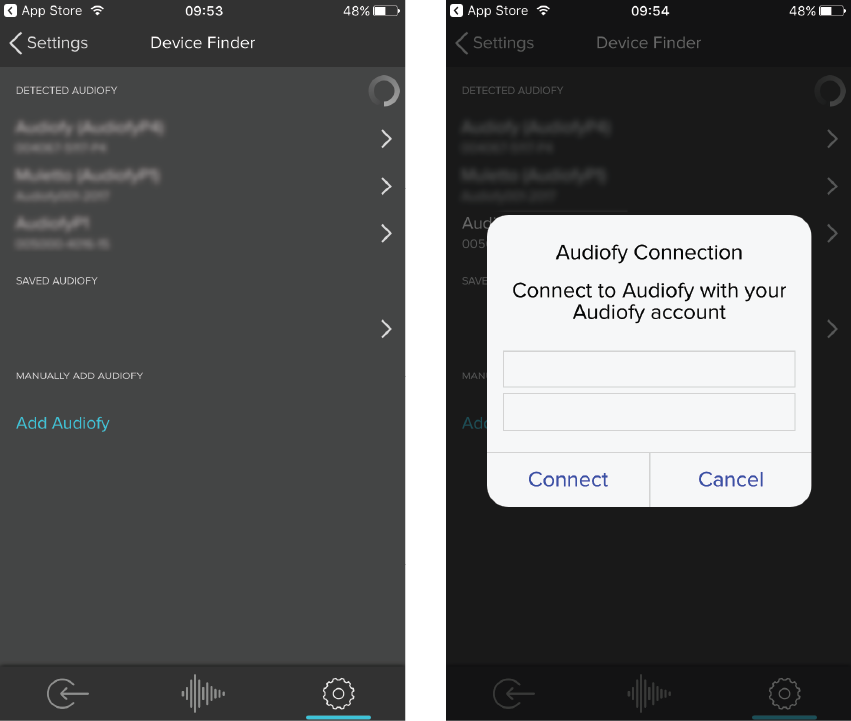The image is a screenshot from a cell phone displaying two distinct screen captures side by side against a completely black background. The left screenshot shows the time as 09:53 with the battery level at 48%. The top of this screen contains a settings icon pointing to the left and the text "Device Finder." Much of the white text on this screen has been blurred, likely for privacy reasons. Notably, there is a circle icon accompanied by the text "Detected Audiophy" and towards the bottom, the option to "Add Audiophy."

The right screenshot, taken at 09:54 with the same battery level of 48%, features a pop-up box stating "Audiophy Connection" with instructions to "Connect to Audiophy with your Audify account." This dialog box offers two options: "Connect" or "Cancel." The overall layout and sequence suggest a step-by-step guide for connecting to the Audiophy service.